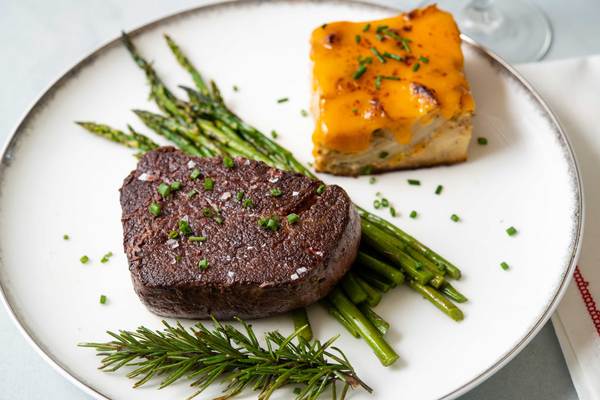In this descriptive photo, a meticulously arranged dish by a chef is presented on a pristine white plate with a subtle gray outline. At the center sits a well-cooked six-ounce steak or filet mignon, dark brown and adorned with finely chopped green onions or chives. The steak is partially resting on a generous bundle of whole, vibrant green asparagus spears, neatly aligned. Below the steak lies a garnish, possibly rosemary or another evergreen herb, adding a touch of freshness to the presentation. In the top right quadrant of the plate, there's a perfectly cut, square piece of an orange cheesy dish, likely a cheese quiche, with a rich, gooey texture, also garnished with a sprinkling of green chives. The setting includes a partial view of a wine glass base in the background and a white cloth napkin with a red border situated to the right, enhancing the overall elegant dining atmosphere. There are no additional elements or text in the image, keeping the focus entirely on the artful presentation of the meal.